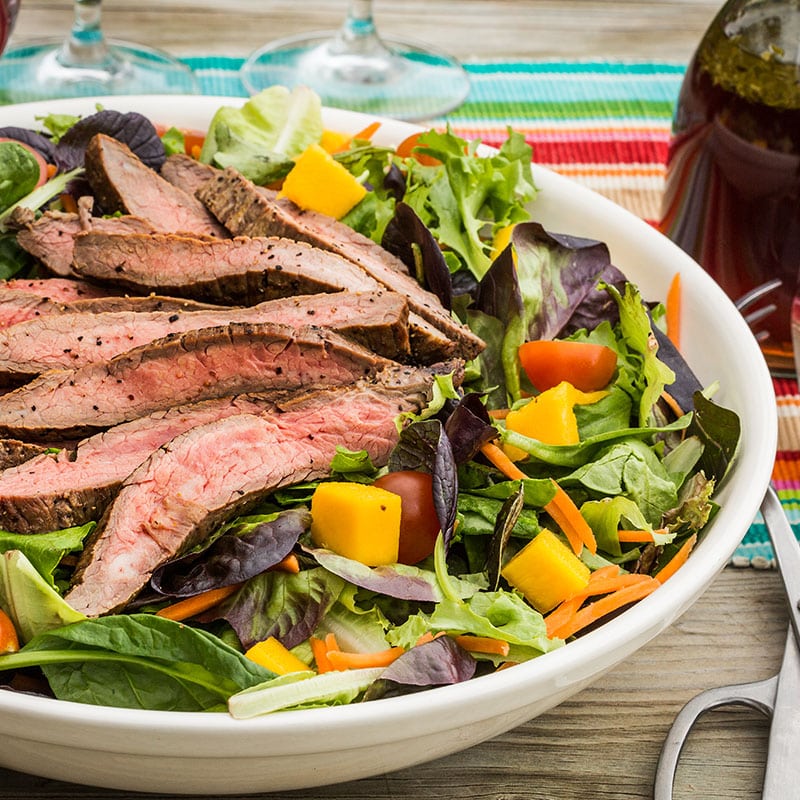This close-up photograph showcases a visually appealing dish set against a wooden table with a rainbow-colored seersucker placemat beneath a white porcelain plate. The centerpiece of the dish features fanned-out, seasoned strips of medium or medium-rare steak, creating an attractive array that narrows toward the center. Below the steak, a vibrant bed of mixed salad greens includes spinach, purple and red lettuce, cherry tomatoes, shredded carrots, yellow peppers or mango, and cheese. The presentation is further enhanced by the presence of two glassware stems, likely from wine glasses, positioned at the front of the plate. Flanking the white plate, on the wooden table, are silver kitchen shears and tongs on the right, and a partially obstructed fork on the left. An additional detail, possibly a reddish vial containing oil or vinegar, can be spotted in the background, enhancing the allure and intricacy of the scene.